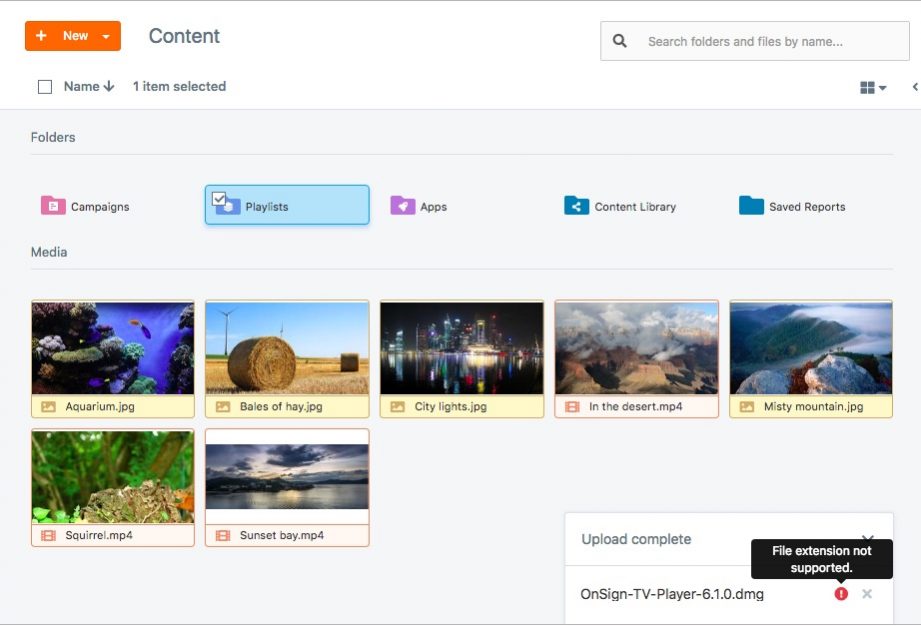This horizontal rectangular image depicts a detailed interface, presumably of a content management system, organized into several sections with various labeled buttons, icons, and file listings.

At the top, there's a thin gray line running horizontally across the image. On the left side of this line, there is a prominent orange rectangular button featuring white text that reads "New," accompanied by a white plus sign to the left and a small pull-down menu to the right. Adjacent to this button, the word "Content" is displayed in blue font. On the right side of this section is a search box.

Moving leftward below the thin line, there's an empty square with the label "Name" next to it and a downward arrow. Adjacent to this, the text "1 item selected" is visible. Several icons are positioned to the right of this text.

The majority of the interface beneath this section rests on a light gray background. In the top-left corner of this gray area, the word "Folders" is prominently displayed. Below this section, different menu items are listed in black font. These include "Campaigns," "Playlists" (which uniquely stands out being highlighted in light blue with a brighter blue outline forming a horizontal rectangle), "Apps," "Content Library," and "Saved Reports." Each of these menu items is accompanied by a relevant icon to their left.

Further down on the left side, the word "Media" is listed. Under this heading, a grid of file thumbnails is displayed in two rows. The first row contains five horizontal rectangular images:
1. "Aquarium.jpg" – an image of an aquarium, labeled in black lettering within a light yellow bar.
2. "Bales of hay.jpg" – an image featuring circular bales of hay, also labeled in black on a yellow bar.
3. "Citylights.jpg" – an image of a city at night with its reflection on the water, labeled similarly.
4. "In the desert.mp4" – an image resembling a canyon with clouds, labeled in white on a muted light bar.
5. "Mistymountain.jpg" – an image of mountains labeled in black on a yellow bar.

The second row contains two items:
1. "Squirrel.mp4" – an imagery of trees and possibly a squirrel, without a yellow label.
2. "Sunsetbay.mp4" – a picture of a sunset, similarly without the yellow label.

At the bottom right, there's a horizontal rectangular area indicating an upload status: "Upload Complete" in light gray with the string "onsign-tv-player-6.1.0.dmg" in black fonts and lowercase. Next to this, a small red circle featuring a white exclamation point and an adjacent flag with the message "File extension not supported" in black with white text notes an error.